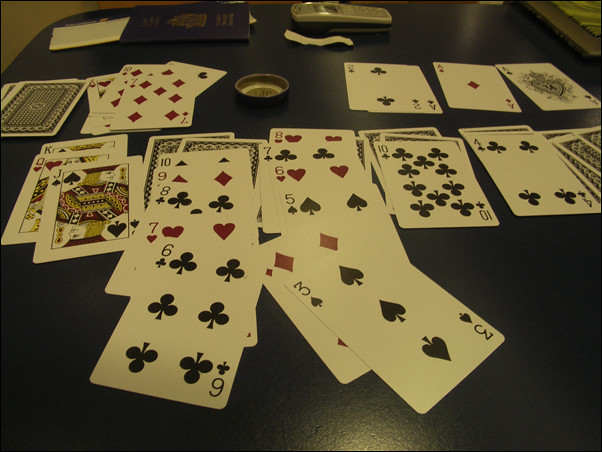The photograph captures an engaging game of solitaire in progress on a dark black table with rounded edges. In the upper left-hand corner, a white envelope lies on its side, topped by a blue passport. Adjacent to this, at the top center, rests a silver non-smartphone alongside a white strip of paper. The top right-hand corner reveals a hint of a piece of furniture, perhaps a table.

The tableau of cards is meticulously arranged. The first deck, likely the stockpile, lies face down. Nearby is the discard pile, currently featuring the ten of diamonds and the seven of diamonds. A cup, possibly used as a lid, sits upright beside these.

The foundation piles, or "castle piles," are clearly visible, with an ace and two of clubs, an ace of diamonds, and an ace of spades in place. The draw cards are stacked in the upper left-hand corner. 

Moving towards the upper right-hand corner, the tableau columns showcase a range of cards:
- The first column: King of spades.
- The second column: Queen of hearts, jack of spades.
- The third column: Ten of spades, nine of diamonds, eight of clubs, seven of hearts, six of clubs.
- The fourth column: Eight of hearts, seven of clubs, six of hearts, five of spades, four of diamonds, three of spades.
- The fifth column: A few cards faced down, followed by the ten of clubs.
- The sixth column: A few cards faced down, followed by the four of clubs.
- The seventh column: Four cards faced down.

The scene is carefully composed, reflecting both the organization of the game and the surrounding elements that add context to this snapshot of a solitaire session.